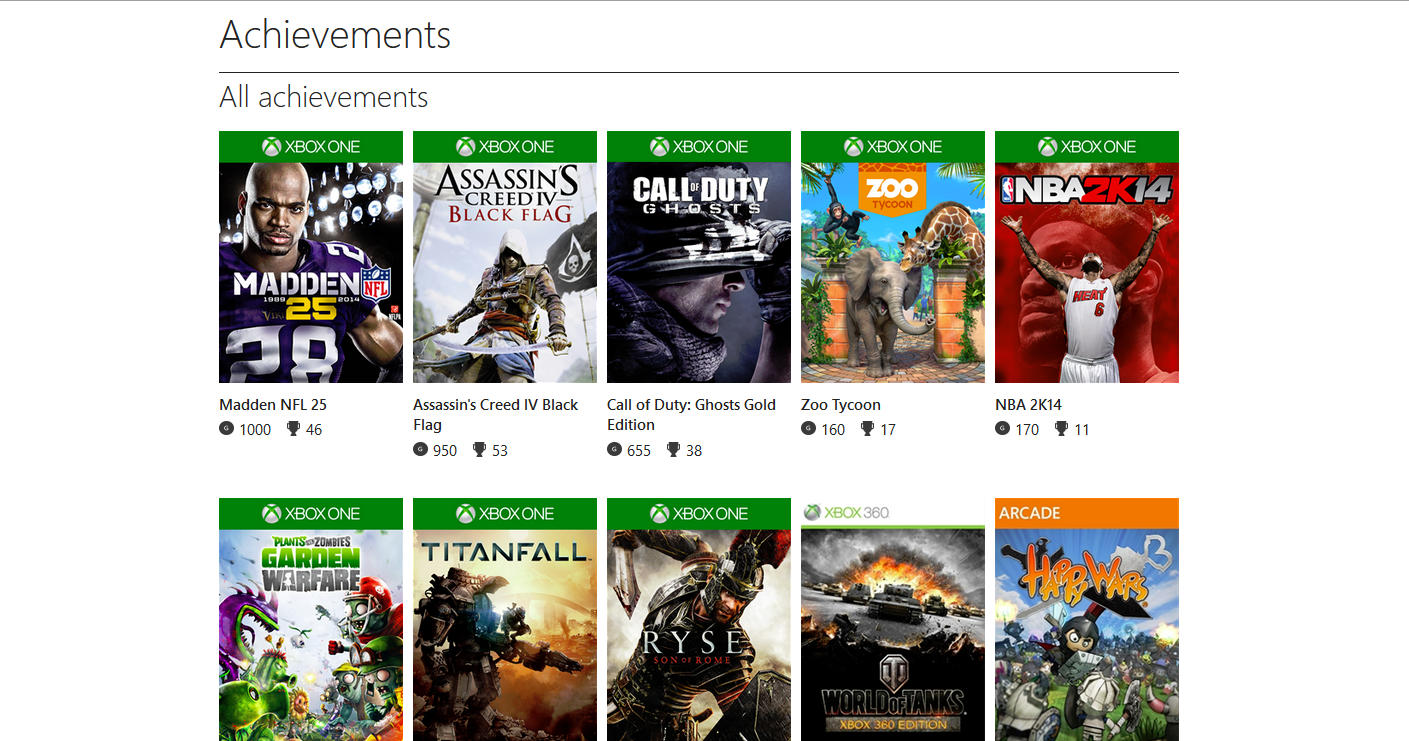This image is a screenshot likely taken from the backend of Xbox Online. At the top, a thin gray line runs across the screen, with "Achievements" prominently labeled in large gray letters at the upper left corner. Below that is another gray line; underneath it, in a lighter gray font, is the text "All Achievements."

The main section of the screenshot features two rows of five Xbox video games each. The top left game in the first row has a green banner with the Xbox logo in white, alongside the text "Xbox One." The first game listed is "Madden NFL 25," showing a score of 1000 next to a trophy icon with the number 46. The second game is "Assassin's Creed IV: Black Flag," displaying a score of 950 and another trophy icon with the number 53. In the center of the row is "Call of Duty: Ghosts Gold Edition" with a score of 655 and a trophy number of 38. Next is "Zoo Tycoon" with a score of 160 and a trophy icon showing 17. The final game in the first row is "NBA 2K14," which has a score of 170 and a trophy number of 11.

The second row also features five games, beginning with three that have a similar green banner at the top with "Xbox One" in white text. Unlike the first row, this one does not display detailed scores or trophy icons for the games. The first game listed is "Plants vs. Zombies: Garden Warfare," followed by "Titanfall," and then what appears to be "RYSE." The fourth game in this row has a white banner with the Xbox logo and "Xbox 360," but the game name is obscured and appears to include the word "War." The final game in this row has an orange banner with "Arcade" in white letters, and the title seems to be "Hair War" or "Har War," though it is not entirely clear.